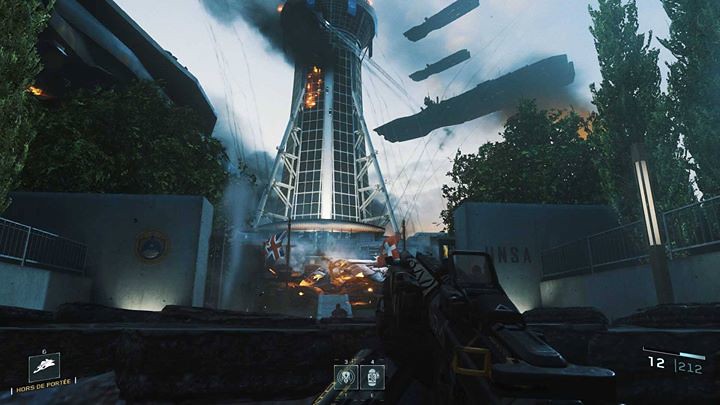The photograph captures a dramatic and intense scene. In the center, a stone wall with an opening reveals a large multi-story tower engulfed in flames. Dark, ominous clouds fill the sky, enhancing the sense of chaos. Silhouetted against this backdrop, several aircraft can be seen flying through the air. A military vehicle is prominently positioned in the foreground. The stone wall features bold lettering on one side that reads "UNCA" and "UNSA," adding an additional layer of intrigue to the image.